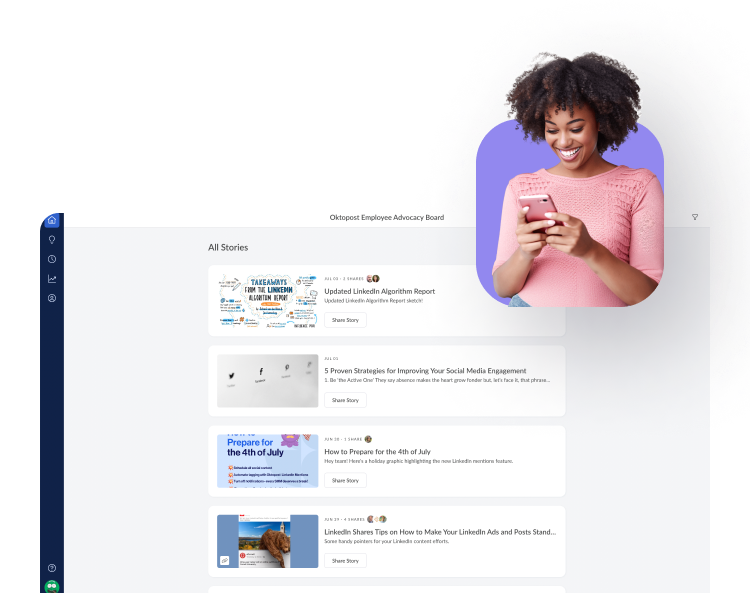In the top right corner, the image features a woman engaged with her cell phone. She is wearing a pink shirt and holds the device, which is encased in a pink cover, with both hands. The woman, who has black hair and a darker skin tone, is smiling against a purple, square-like background. 

On the left side of the image, set against a dark blue background, there are seven icons arranged vertically—five at the top and two at the bottom. Adjacent to this section is a light gray square displaying the title "All Stories" at the top in gray text. Below the title are four white rectangles, each containing different links. The links include:

1. "Updated LinkedIn Algorithm Report"
2. "Five Proven Strategies for Improving Your Social Media Engagement"
3. "How to Prepare for the 4th of July"
4. "LinkedIn Shares Tips on How to Make Your LinkedIn Ads and Posts Stand Out"

Each link is accompanied by an image to its left, and the background of this section is white. At the very top of the overall image, the text reads, "Okay to Post Employee Advocacy Board."